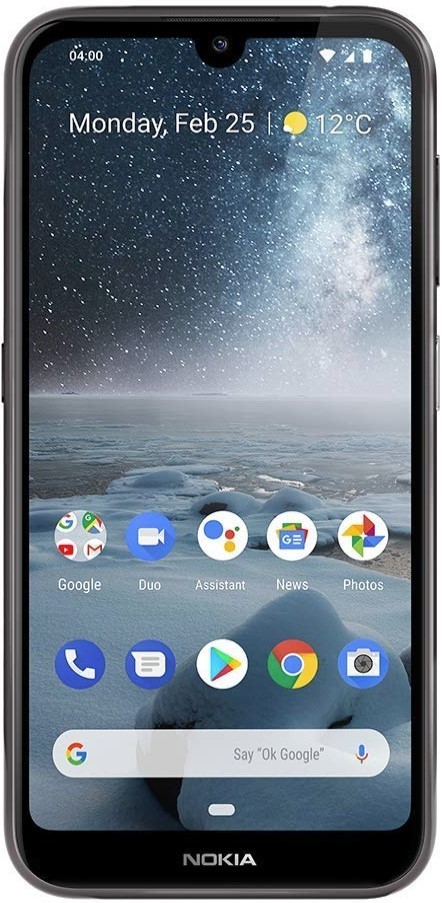A detailed photographic image showcases a Nokia mobile device with a silver-edged, rectangular design and a black rim outline. The device's screen is illuminated, displaying various app icons including Google, Duo, Assistant, News, and Photos. The soft touch buttons are visible on each side. It's precisely four o'clock, as noted by the device. The camera is centered on the front top of the device alongside icons indicating Wi-Fi connectivity, carrier signal, and battery life. The date and time at the top read "Monday, February 25th" and the temperature is a chilly 12 degrees Celsius. The background image features an Arctic-like scene with glaciers covered in ice. Above the icy landscape, the night sky is adorned with the Milky Way and a multitude of stars, suggesting minimal cloud coverage and clear visibility.